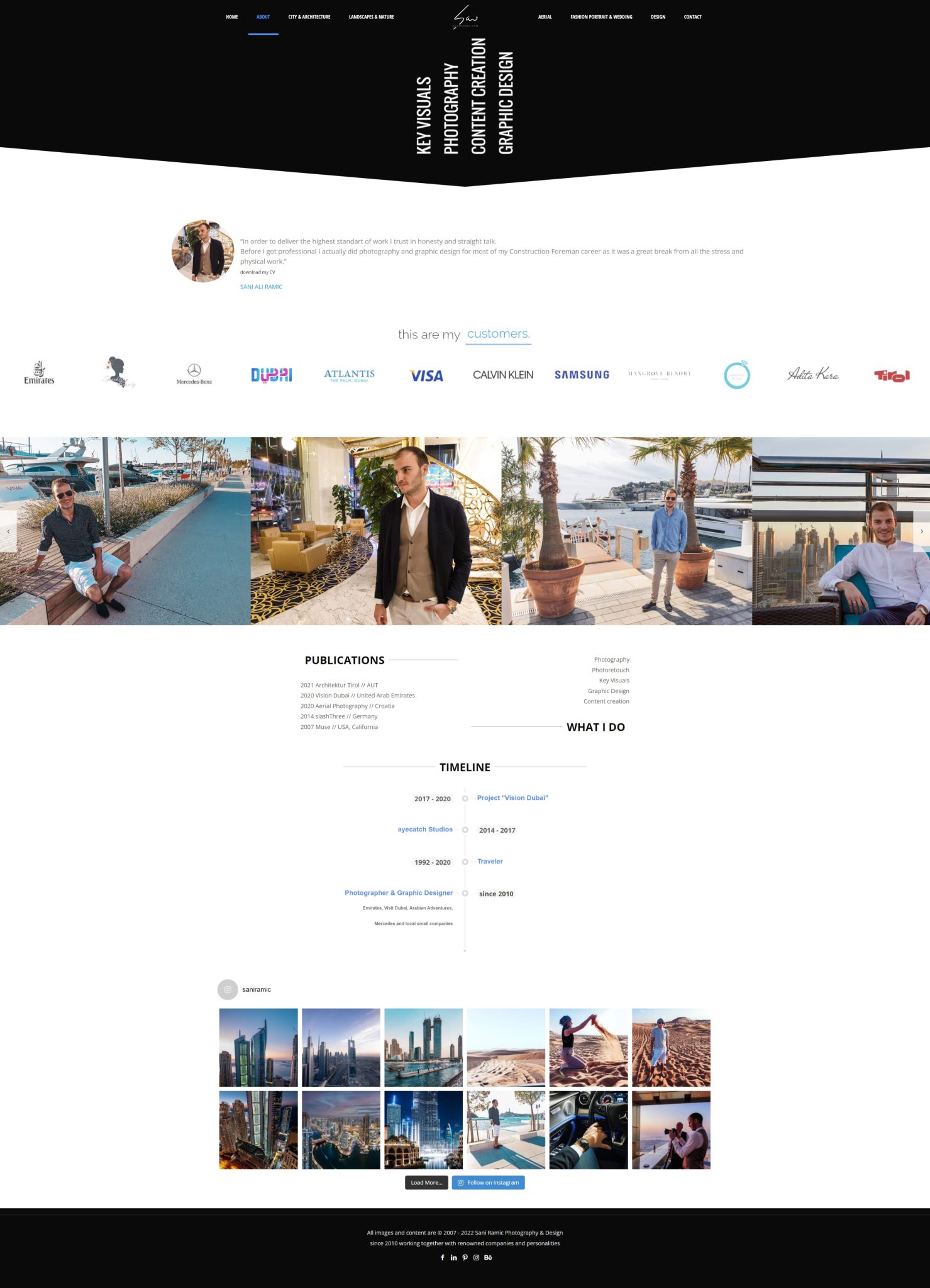Screenshot of a professional portfolio website with a sleek, modern design. At the very top, a black navigation bar spans the width of the page, featuring a centered set of white text links. The second link is highlighted in blue, indicating the current page. Positioned in between the links is a logo.

Directly below the navigation bar, sideways-aligned topics such as Key Visuals, Photography, Content Creation, and Graphic Design are listed. Beneath these topics, there's a section presumably introducing the website owner. This section includes a small circular photograph on a white background accompanied by a brief biography centered on the page. 

Further down, there’s a heading that reads "My Customers" with the word "Customers" underlined in blue. A horizontal row of logos representing various companies, including Visa, Calvin Klein, and Samsung, follows this heading.

Below this, the website displays four photographs of the owner in various settings, with arrows that suggest additional images can be scrolled through. Continuing downward, there's a list of publications followed by a section titled "What I Do" along with a timeline of the owner’s career or major projects.

At the bottom of the page, an Instagram feed is showcased, complemented by two buttons – one black and one blue. Finally, the footer of the website features another black bar with white text and links.